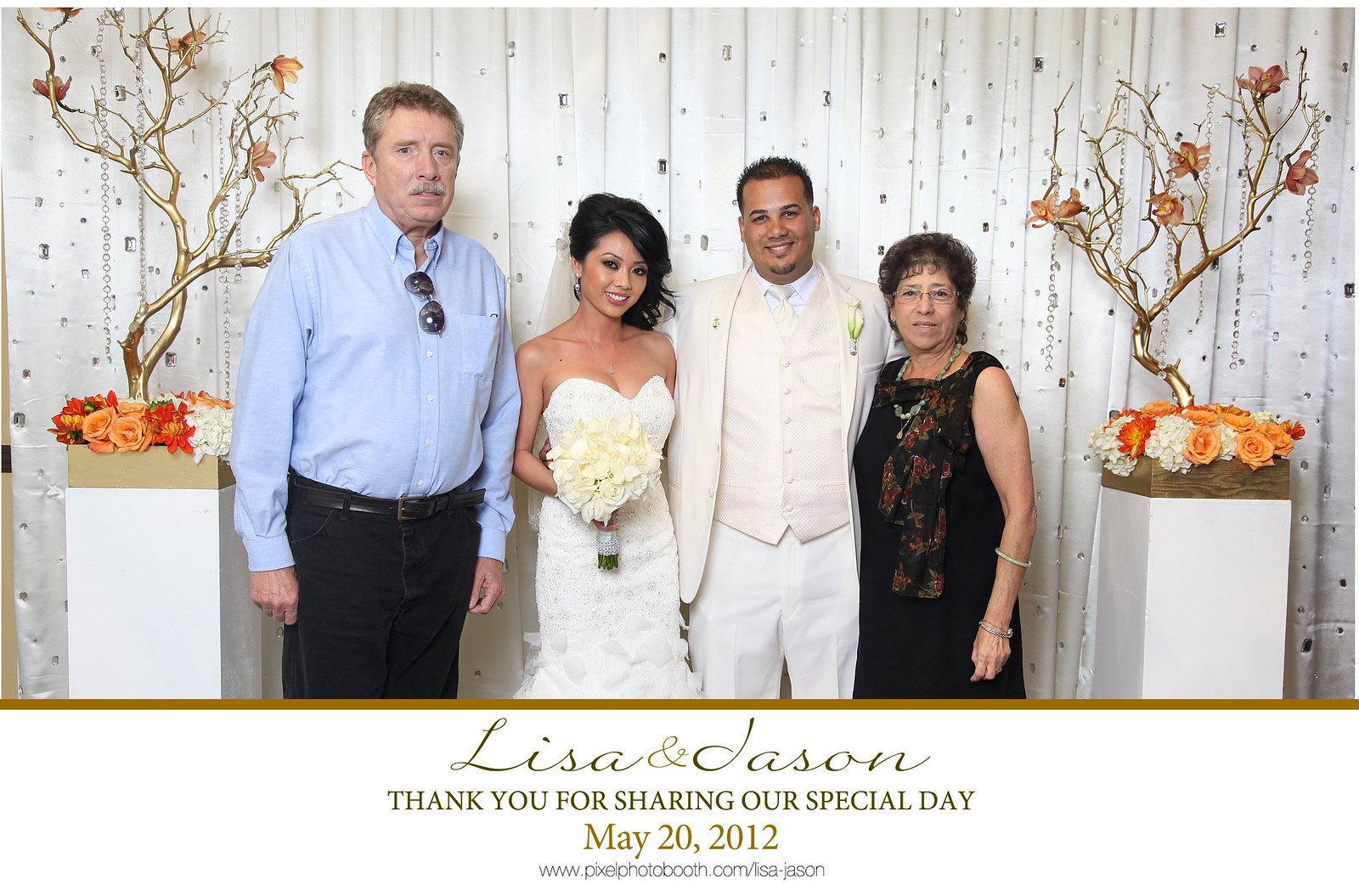In this professionally shot wedding thank you postcard, four individuals stand in front of a white curtain adorned with gold designs. Centrally positioned are the newlyweds: a young groom in a white tuxedo with a flower on his lapel, and a bride with black hair, a veil, and a sleeveless white wedding dress, carrying a white bouquet of roses. Flanking the couple are the likely parents. To the right of the bride stands an older man with graying hair, a gray mustache, a blue long-sleeved shirt, and black pants. To the left of the groom is an older woman with graying hair, wearing a sleeveless black dress. Each parent stands beside a pedestal with a floral arrangement and a gold-accented tree. The card's message underneath reads: "Lisa and Jason, thank you for sharing our special day, May 20, 2012," alongside the website www.pixiefotoboot.com.